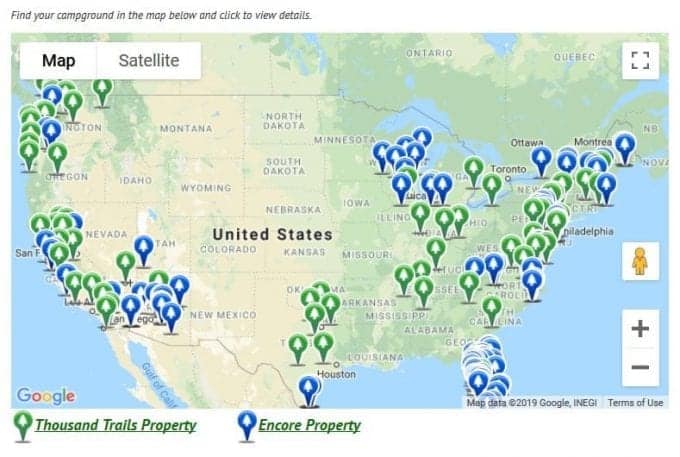This low-resolution map of the United States illustrates various campgrounds marked with location pins. According to the legend, the green pins indicate "Thousand Trails Property" while the blue pins denote "Encore Property." The map is an interactive Google Map, allowing users to zoom in and out, switch between map and satellite views, and access street views. The layout is at a high-level view, showcasing the outlines and names of the states. The location pins are predominantly clustered around the West Coast, East Coast, and the northern Midwest, with a few scattered in Texas. Notably, there are sparse or no pins across the Plains States and the Mountain West. The caption reads: "Find your campground on the map below and click to view details."